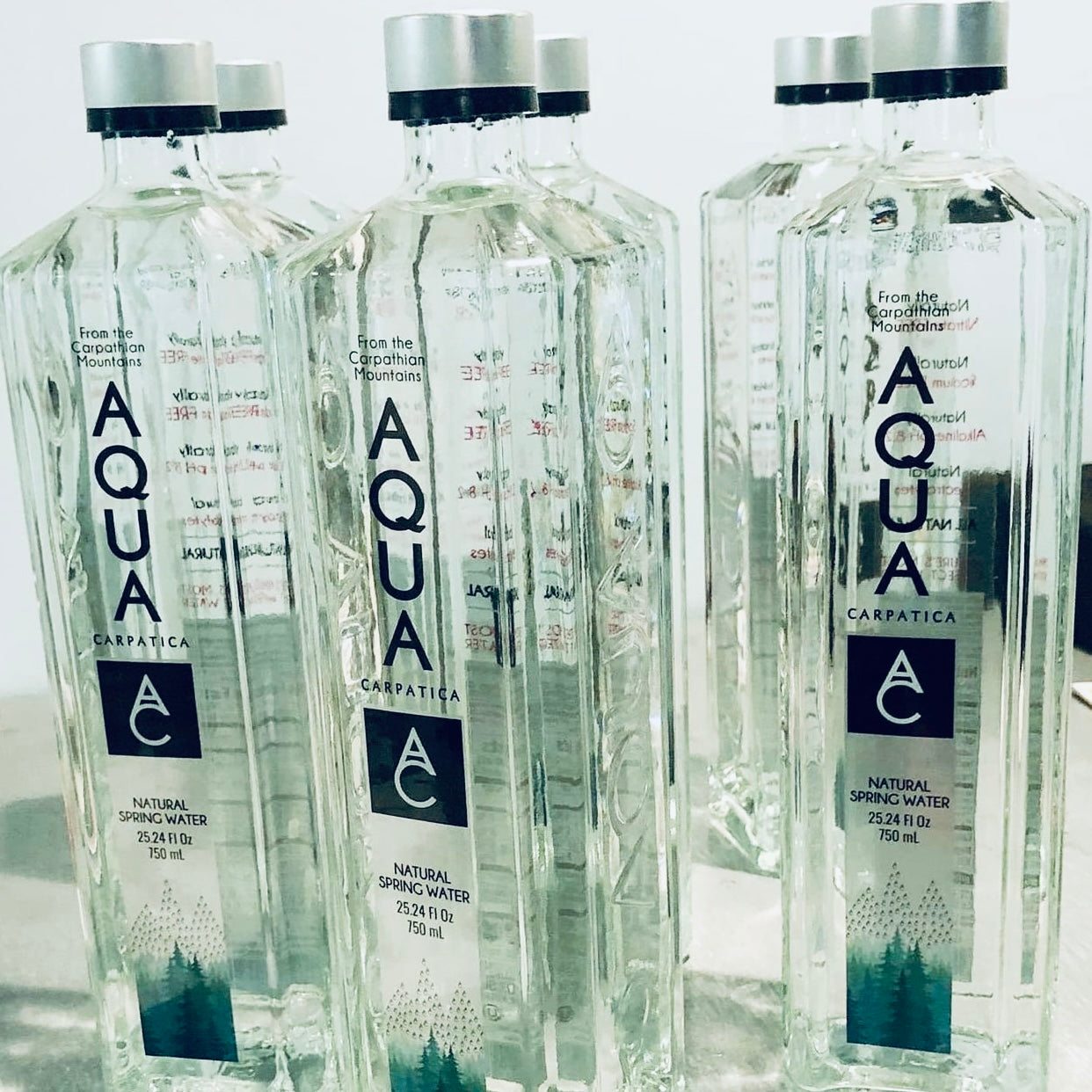This photograph features an elegant arrangement of six clear Aqua Carpathica natural spring water bottles, each holding 25.24 fluid ounces (750 milliliters), standing atop a white background. The tall, narrow, and square-shaped glass bottles are crowned with silver caps, accented by a subtle black band. Prominently, the labels display "From the Carpathian Mountains" in fine font at the top, followed by the name "Aqua" printed vertically in bold black letters. Beneath, "Carpathica" is written in smaller font. A distinct black logo, resembling an 'A' on top of a 'C', is placed below the brand name. The label, which is clear like the bottle, reveals an artistic depiction of white mountain peaks surrounded by green pine trees and black droplets shaped like trees, emphasizing the pure origin of the water from the Carpathian Mountains. The bottles are organized in three columns, with two bottles in each column, creating a visually appealing presentation.